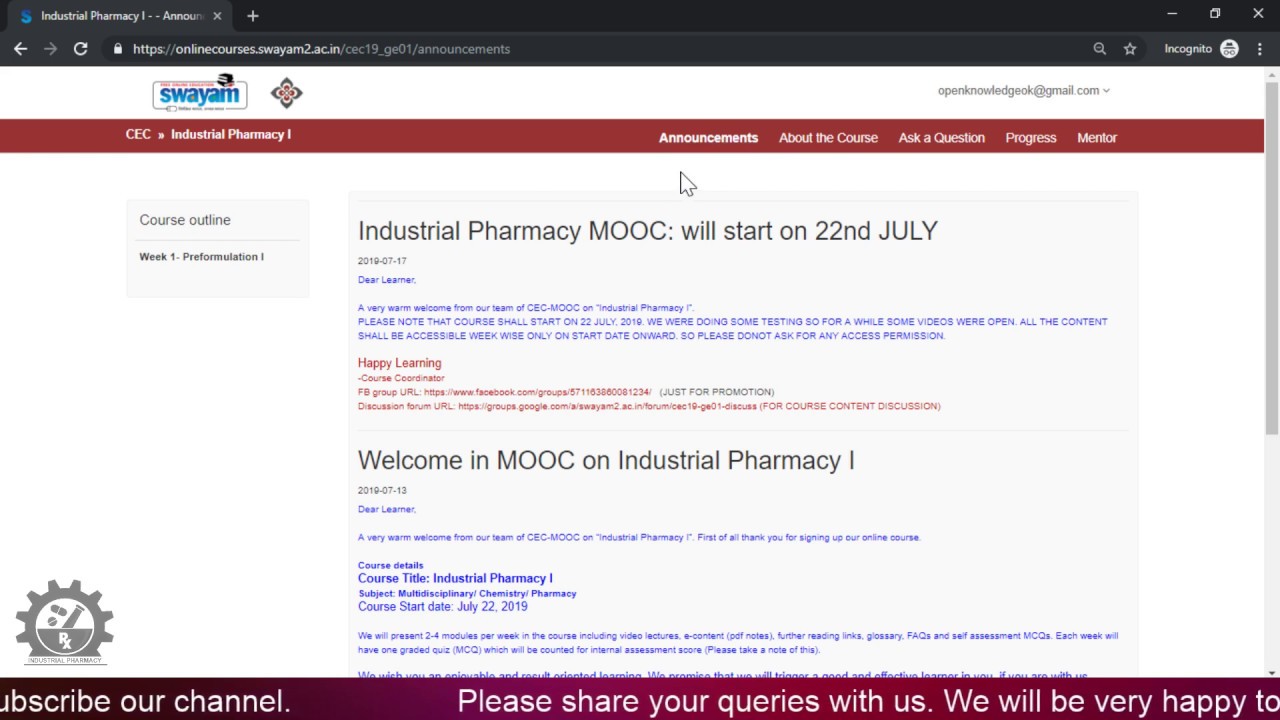The image displays a browser window open to the announcements page of an online course platform, indicated by the web address `https://onlinecourses.swayam2.ac.in/CEC19_GE01/announcements` visible in the address bar. In the upper-left corner, the page features the NAS logo. The browser interface includes standard navigation buttons, such as the back arrow, forward arrow, and refresh icon. Prominently on the page, there is a distinctive S-W-A-Y-A-M logo resembling a license plate, under which the title "CEC Industrial Pharmacy" is displayed. The main section of the webpage highlights the course outline for "Industrial Pharmacy MOOC."